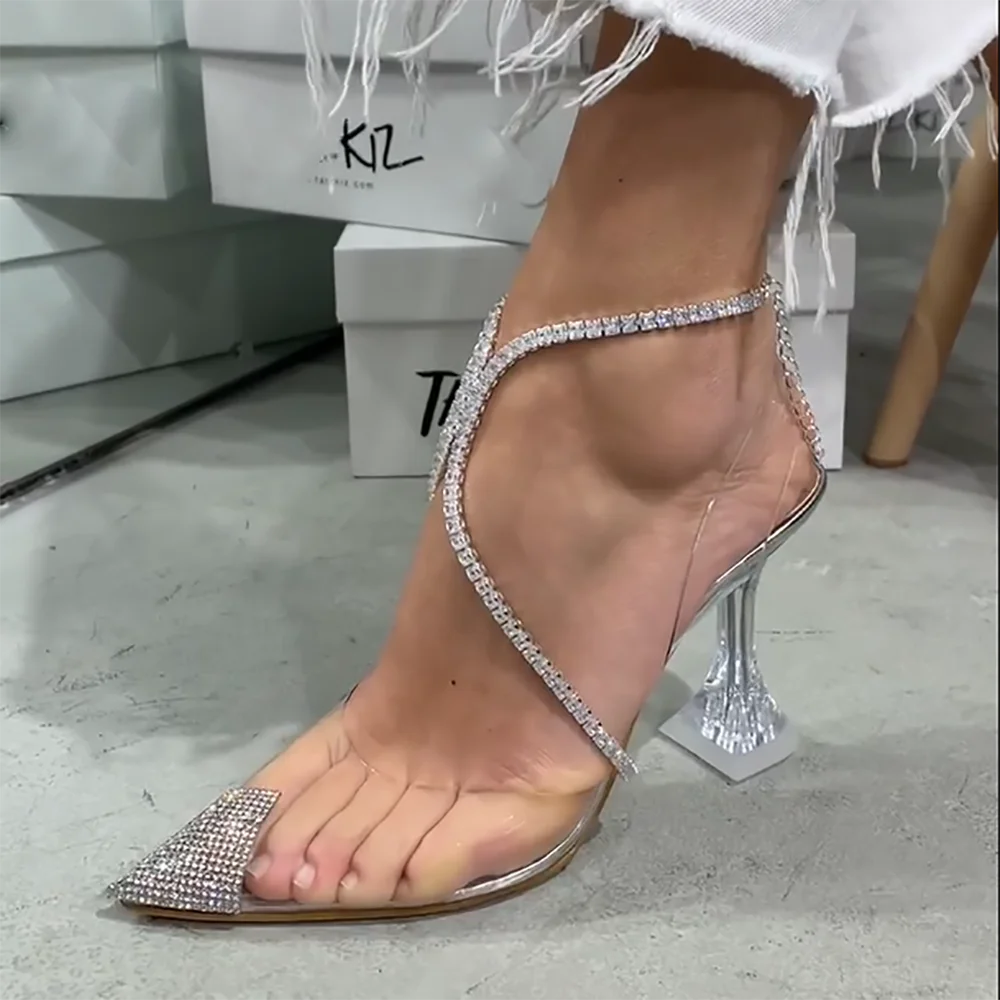The image depicts a close-up of a woman's left foot adorned in an elegant high heel shoe. The footwear is characterized by an open-toe design, although the big toe is covered by a pointed section embellished with glittery rhinestones or resin jewels. The remainder of the toes are encased in a transparent plastic that molds around them. The shoe features straps that form an X over the top of the foot and wrap around the ankle, also adorned with sparkling, diamond-like gemstones. The high heel is made of a translucent material, resembling glass or crystal, offering a refined and delicate appearance. For added stability, thin, almost invisible lines akin to fishing wire extend from the back of the ankle to the mid-foot area. The sole of the shoe is brown, and the backdrop includes stacked white shoe boxes labeled with "KIZ" in black lettering. The wearer is standing on a gray concrete pad and is dressed in frayed white pants that reach down to the cuff of the ankle.